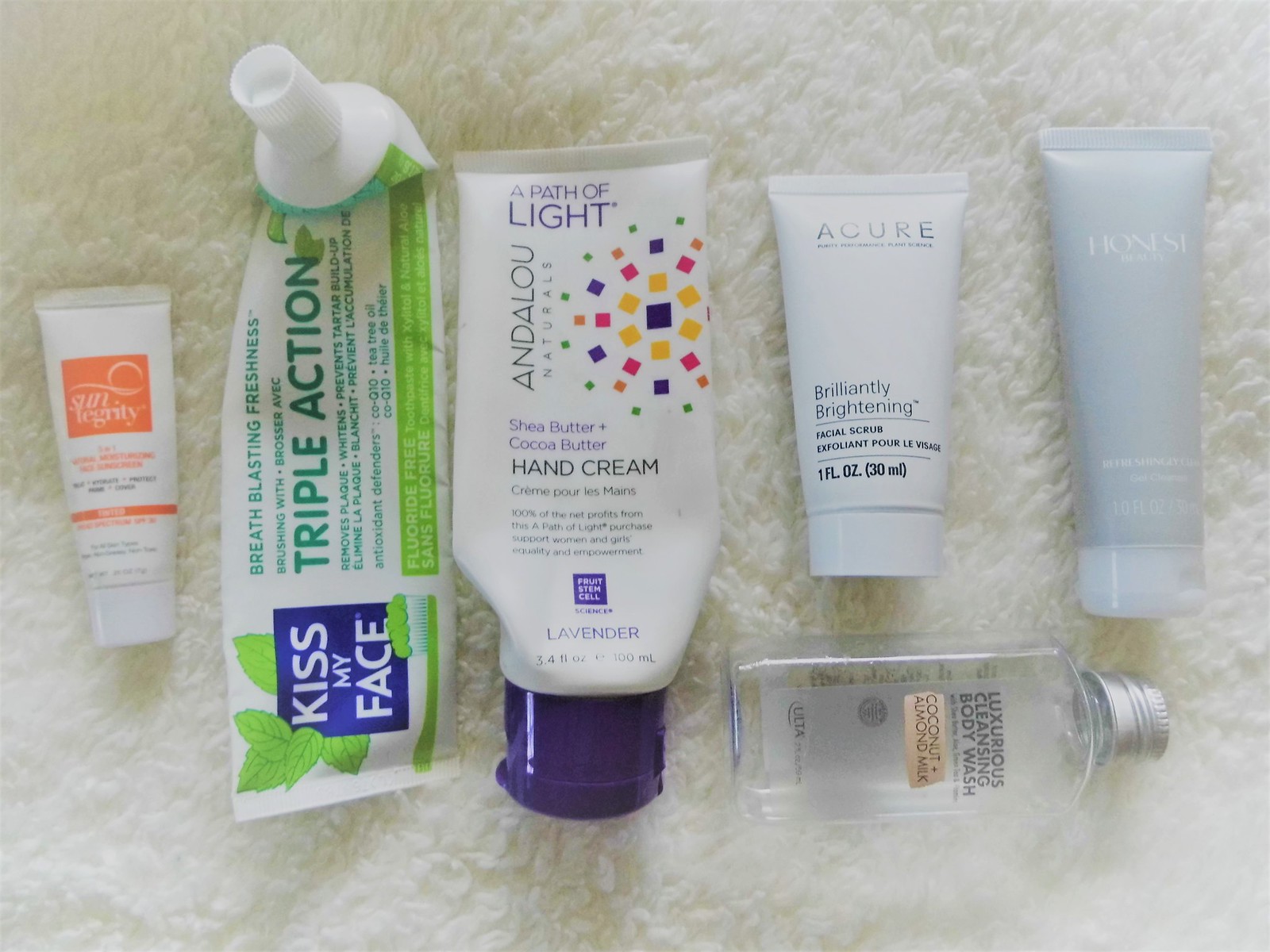In the image, a variety of skincare products are meticulously arranged on a soft, white, fluffy surface that could be either a towel or blanket. The fabric's fuzzy texture creates a cozy and inviting backdrop for the items. There are six distinct products, each with unique characteristics.

1. On the far left, there is a small squeeze tube that appears to be a sunscreen from the brand Suntegrity. The tube is predominantly white with a coral or salmon-colored design and features a screw-on cap. 

2. Next to it is a nearly empty toothpaste tube from the brand Kiss My Face. This product has a blue label with "Kiss My Face" written in white lettering and mint leaf illustrations. It boasts "Triple Action" and "Breath Blasting Freshness," along with an image of a green toothbrush with green toothpaste on it.

3. The third item is a differently styled squeeze tube with a blue screw-on flip cap. This product is from Andalou Naturals and is labeled "Path of Light." It features a vibrant confetti-like flower design and contains Shea Butter and Cocoa Butter Hand Cream with a lavender scent. The label is bilingual, also displaying the product name in French.

4. The fourth product is a small, white squeeze tube from Acure. It holds one fluid ounce of "Brilliantly Brightening Facial Scrub," with additional labeling in French.

5. Fifth in line is a tube from the Honest Company. This tube is predominantly white with pale grey accents and has a translucent flip cap. The exact details and product name are not entirely visible.

6. The final item is a small bottle, possibly glass or plastic, with a metal screw-on cap. Lying on its side, it reveals the label "Luxurious Cleansing Body Wash," featuring a coconut and almond scent. This compact bottle appears to contain no more than an ounce or two of the product.

Each product stands out against the soft, fluffy background, creating a visually appealing arrangement of skincare essentials.